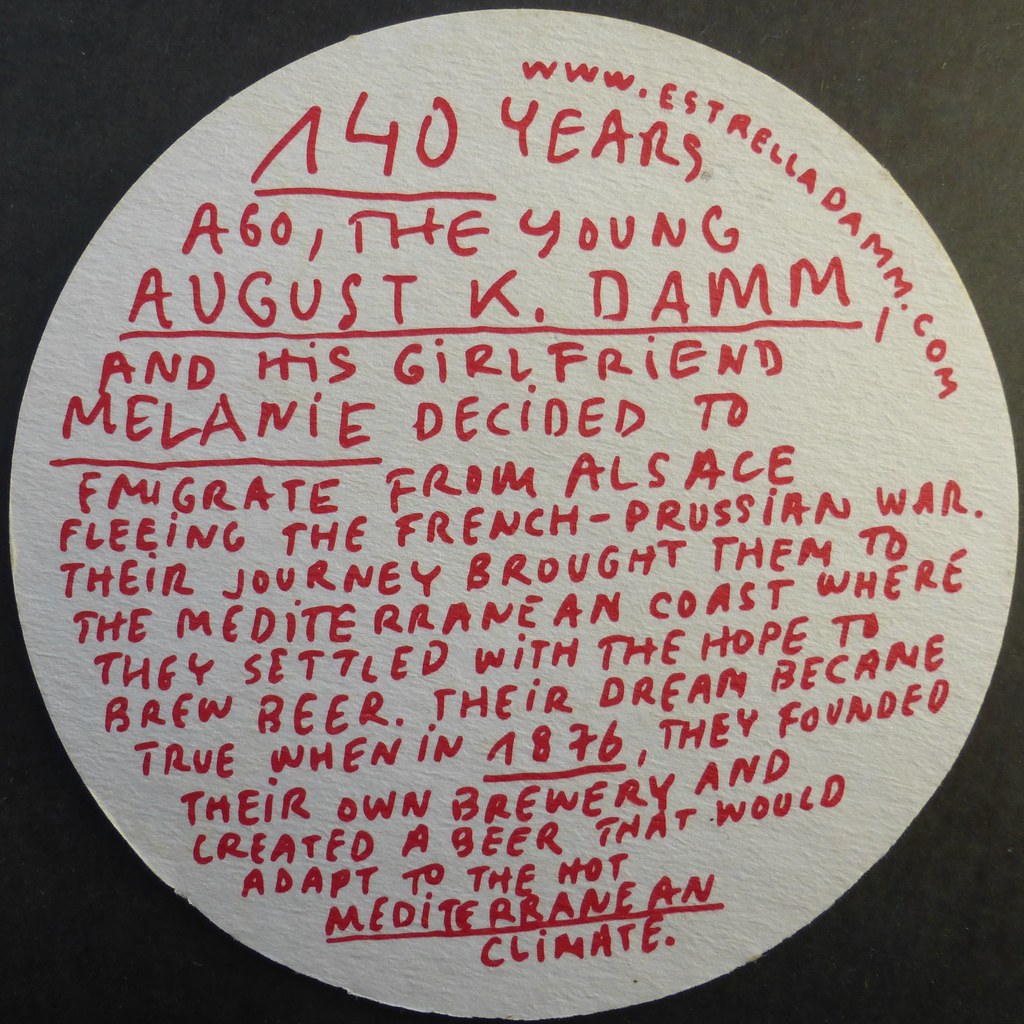The image features a black background with a large white, textured circle that touches the top, bottom, left, and right edges of the image, almost entirely covering the black backdrop. Within this circle, there is red handwritten text in capital letters that follows a circular motion along the perimeter, with additional text written straight across the center. The text reads "www.estrelladam.com" in an arc shape on the upper right-hand side. The main body of the text narrates the story: "40 years ago, the young August K. Dam and his girlfriend Melanie decided to emigrate from Alsace, fleeing the French-Prussian War. Their journey brought them to the Mediterranean coast where they settled with the hope to brew beer. Their dream came true in 1876 when they founded their own brewery and created a beer that would adapt to the hot Mediterranean climate." Certain phrases such as "August K. Dam", "Melanie", "1876", and "Mediterranean climate" are underlined for emphasis.